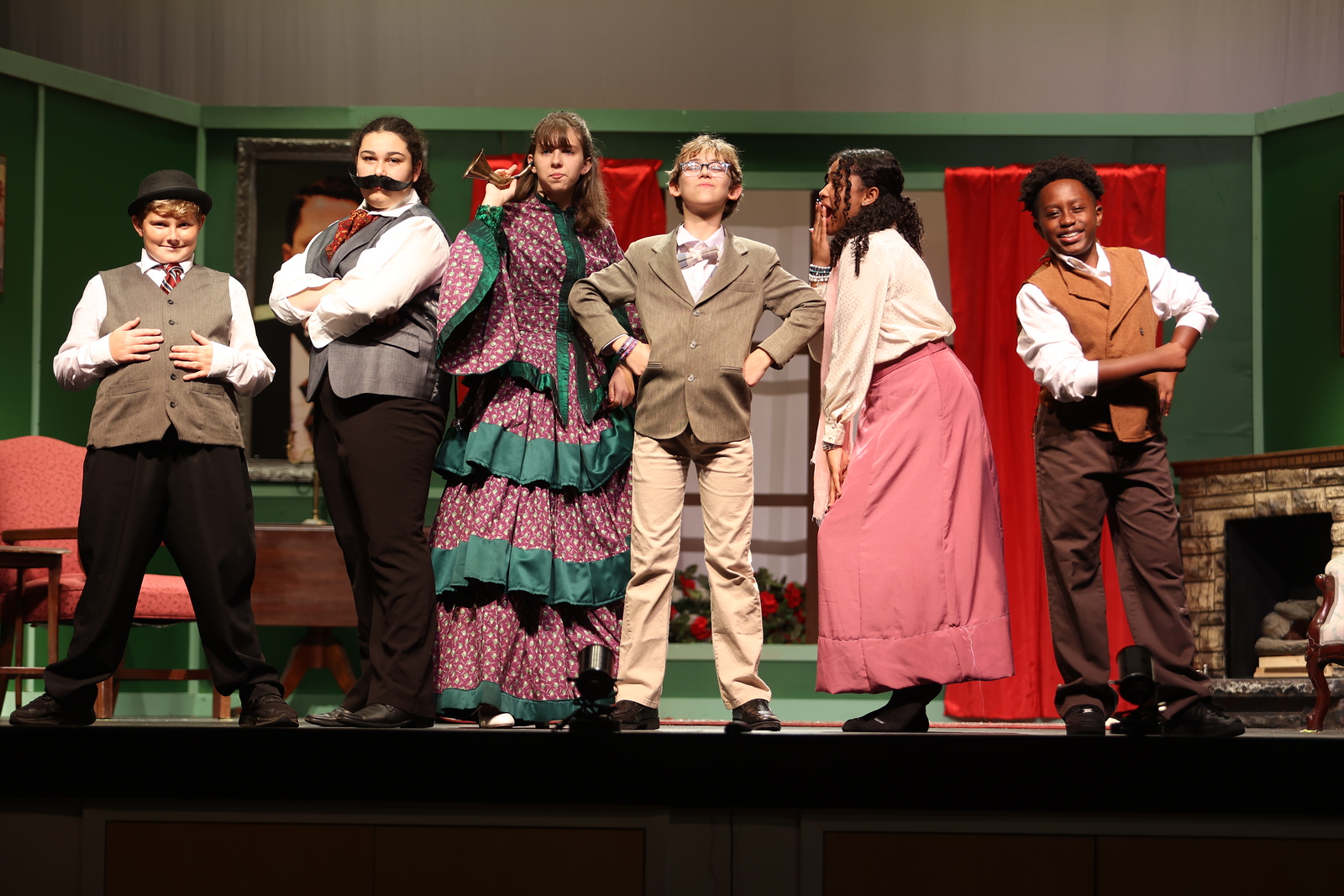This image portrays six young individuals on stage, seemingly during a theatrical performance or rehearsal set in the late 19th century. They are dressed in elaborate, old-fashioned costumes that feature long ruffled skirts for the girls and handlebar mustaches for some of the boys, designed to make them appear older. A prominent feature includes a young boy at the center wearing glasses, a tan jacket with shoulder pads, a tan bowtie, a white collared shirt, and tan pants. To his left stands a taller girl in a purple dress with white dots and green trim, holding an old-fashioned ear horn. Further to the left, another girl wears a fake mustache, a long-sleeve white shirt, a gray vest, and black pants. Next to her is a boy in a white long-sleeve shirt, lighter colored vest, tie, black hat, and black pants. On the far right, a child in a brown vest and dark brown pants rolls up the sleeves of his white shirt. Beside him, a girl in an off-white long-sleeve shirt and a long pink skirt faces towards the boy in the center. The background features red curtains and a green-toned setting with a model of a fireplace in the lower right corner of the stage, adding to the period ambience of the scene. A black horizontal bar is visible at the bottom, possibly indicating the edge of the stage, where the young performers are standing.